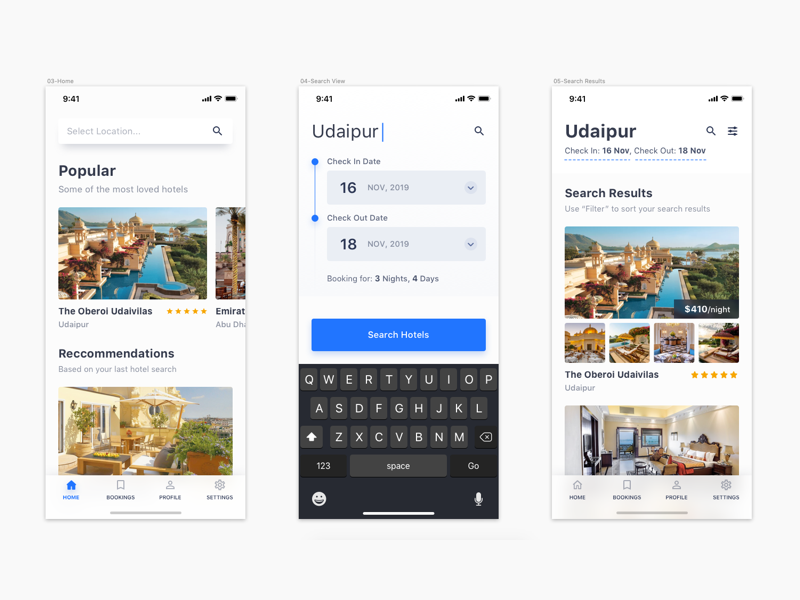This detailed caption describes a collage of three screenshots from the Airbnb app on an iPhone, showcasing a step-by-step guide on how to use the app:

---

**Image Collage of Airbnb App Screenshots: Step-by-Step Guide**

The collage features three images side by side, each exhibiting different sections of the Airbnb app on an iPhone, along with small, descriptive headings in the top left corner of each screenshot.

1. **03 Home:**
   - The background of this screenshot is white.
   - At the very top, a search location bar is prominently displayed.
   - Below the search bar, there's a "Popular" section listing popular destinations or listings, followed by a "Recommendations" section.
   - At the bottom of the screen, four navigation options are aligned side by side: Home, Bookings, Profile, and Settings.

2. **04 Search View:**
   - The top of this screenshot shows the destination "Udaipur."
   - Options to select the check-in and check-out dates are displayed, with the dates chosen being November 16, 2019, for check-in and November 18, 2019, for check-out.
   - Below the dates, it mentions "Booking for three nights and four days."
   - A blue "Search Hotels" button is at the bottom of the view, alongside the device's keyboard.

3. **05 Search Results:**
   - Again, the top of this screenshot features the destination "Udaipur" with the selected check-in and check-out dates.
   - Under the search results section, available hotels or places are listed.
   - The first result is the "Oberoi Uday Vilas," presented with a five-star rating, a carousel view of images, and a price tag of $410 per night.
   - A second listing is also visible, although its name is not shown in this portion of the screenshot.

These images collectively illustrate a user navigating through the Airbnb app to search for hotels in Udaipur, showcasing various functionalities and user interface elements of the app.